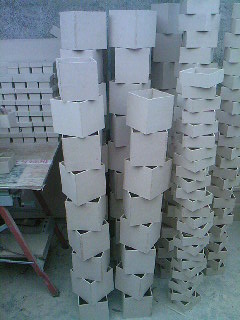The image depicts a room filled predominantly with stacks of variously sized gray boxes, primarily used for filing paper, arranged in several neat columns and rows in the background. The boxes, many of which are empty, occupy the majority of the photograph. They include medium-sized square boxes and shorter, similarly wide ones, giving a structured but somewhat haphazard appearance as some stacks in the foreground are irregularly aligned, with boxes placed diagonally on top of each other. To the left, there is a red portable table with sawhorse legs, potentially holding a piece of machinery like a sewing machine. Behind this table, additional stacks of smaller boxes, possibly jewelry-sized, can be seen. The room features a grayish-blue wall and a cement floor, adding to the minimalist and utilitarian aesthetic.